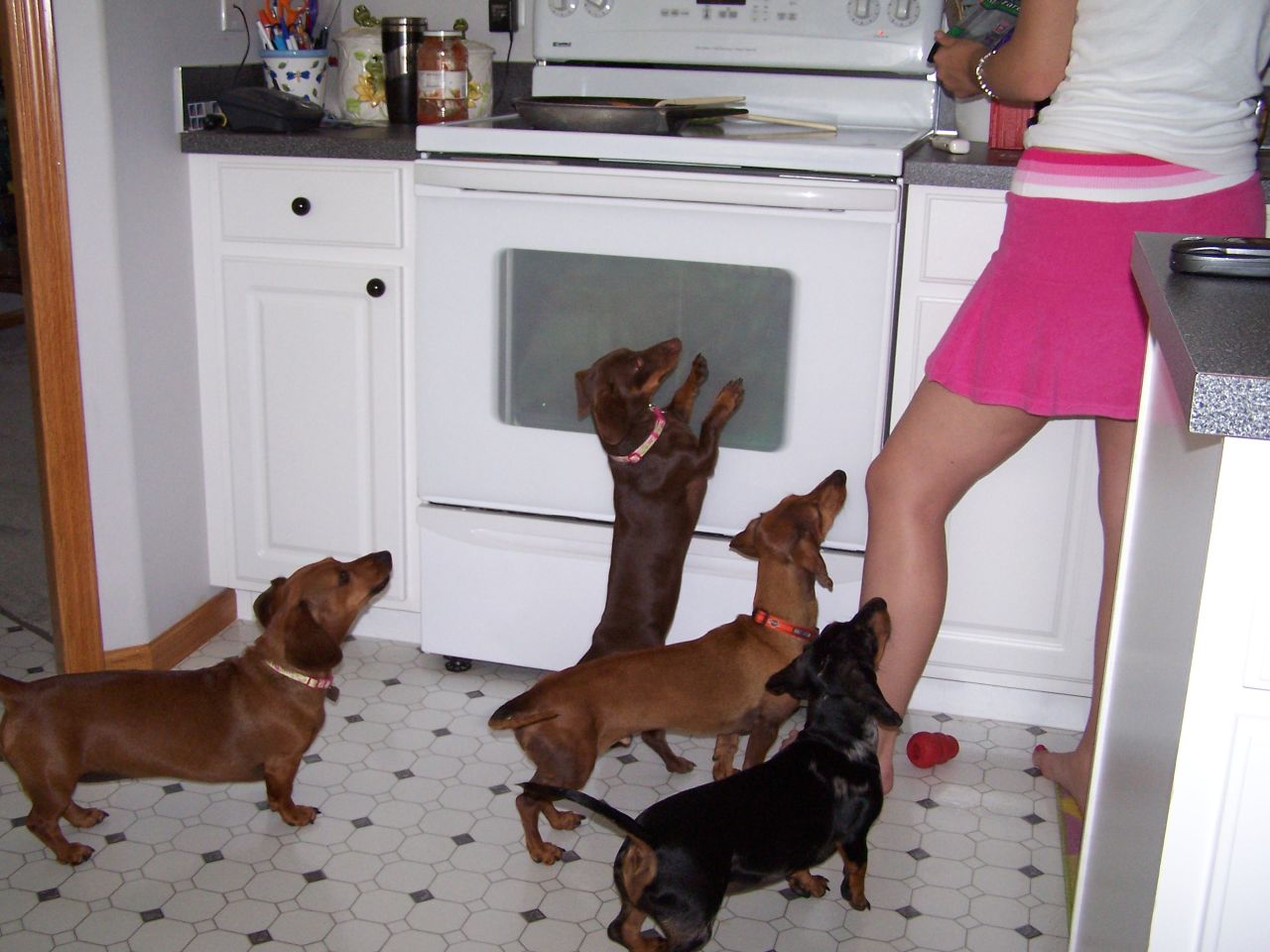In this vibrant kitchen scene, a light-skinned woman is seated near the gray marble kitchen counters, wearing a chic ensemble of a hot pink dress with alternating white and pink stripes, and a crisp white shirt. She accessorizes with a silver bracelet on her left arm and sports red-painted toenails. Surrounding her are four eager dachshunds: one chocolate brown with a pink collar and olive, another chocolate brown with a red collar and black clasp, a black one with chocolate brown markings on its face, feet, and rear, and another chocolate brown one with lighter patches near its eyes and mouth. 

The kitchen's white linoleum floor features a distinctive repeating pattern of white hexagonal shapes interspersed with black diamonds. White cabinetry with black handles, a white stove with a gray pan and a beige spatula, and an assortment of kitchen items such as a jar of Prego, a silver thermos, and a cup filled with scissors and pens adorn the backdrop. The dogs, fixated on the woman, seem to be begging for treats she might be holding. A small lighter, a ceramic white cookie jar, and a red toy on the floor add to the cozy domestic atmosphere. The scene captures a delightful and bustling moment in a modern, homely kitchen.